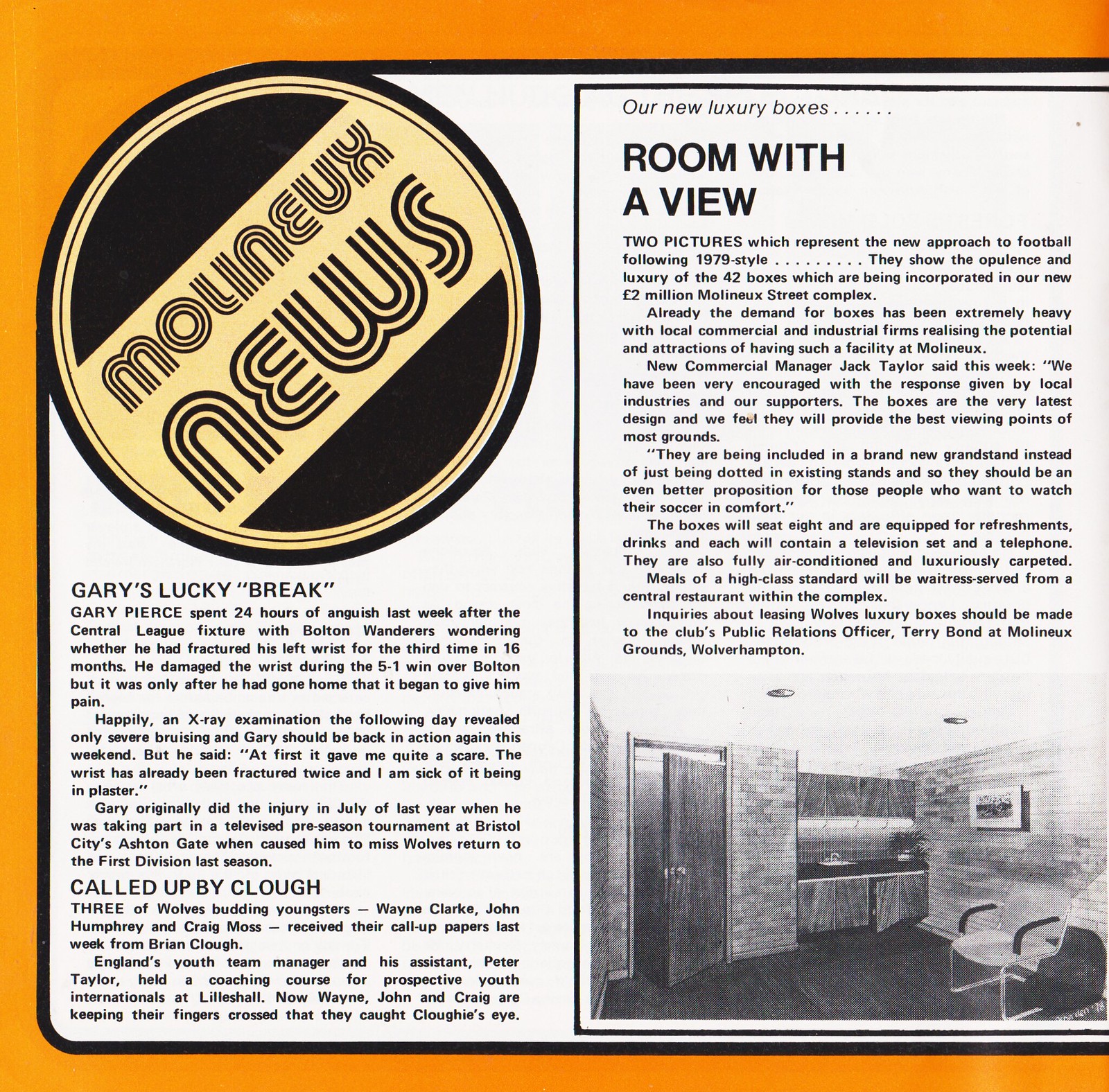The image appears to be a page from an old magazine or newspaper, characterized by a worn, nostalgic aesthetic. It is bordered on three sides—top, left, and bottom—by a bright orange frame, which is conspicuously absent on the right edge as though the border has been cut off. At the top left corner of the central white box, there is a bold, eye-catching black circle with a cream-colored strip across its center containing the stylized retro text "Molyneux News."

Below this heading, the section titled "Gary's Lucky Break" is prominently displayed in black lettering, followed by a detailed paragraph. Near the bottom of this section is another subtitle, "Called up by Clough," accompanied by additional explanatory text. Adjacent to this on the right, there is another segmented section, divided vertically by a black line. The titles here read "Our New Luxury Boxes" and "Room with a View," the latter being in large black font. Under this headline is another comprehensive paragraph. This rightmost section also contains a grainy, low-resolution black-and-white photograph of a room featuring dark flooring, brick walls, a chair in the right corner, and a closet on the left side.